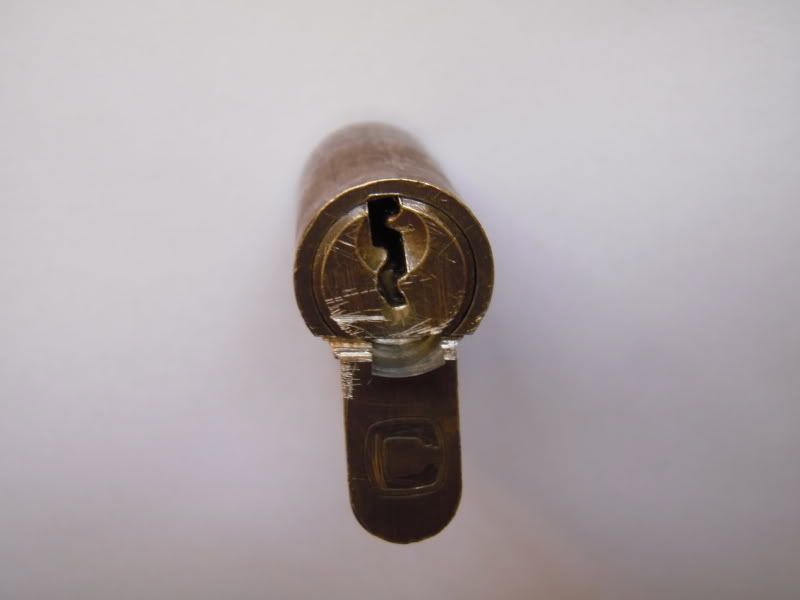The image depicts a brown log with a cylindrical keyhole in the center, highlighted by a golden area around it. The background is gray, and the log is prominently centered. The image features a watermark comprising a white, semi-transparent spiral logo to the left of the log. To the right of this logo, the words "photobucket" appear in a nearly opaque white text, stretching across the log. Below "photobucket," a transparent gray strip bears the slogan, "protect more of your memories for less!" in darker gray letters. This layout suggests that the image functions as an advertisement conveying security, likely for Photobucket’s services.